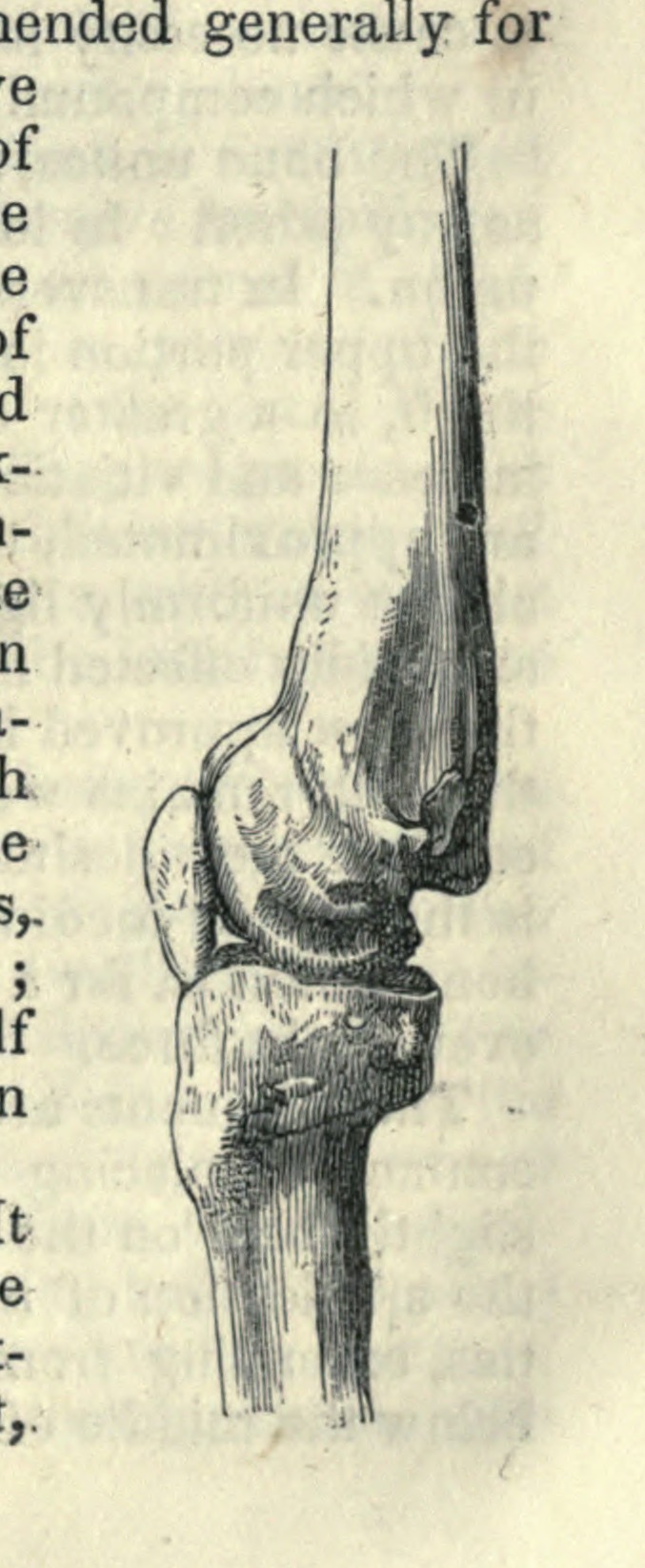This black-and-white, hand-drawn illustration, likely sourced from a textbook, depicts the knee joint in intricate detail, showing the patella, femur, tibia, and fibula. The drawing appears on a yellow-tinged, long rectangular piece of paper, and features meticulous shading that enhances its realism. At the top of the piece, the partial text "E-N-D-E-D" and "generally for" is visible, suggesting it was cut from a larger page. Along the left edge, remnants of letters hint at adjacent paragraphs from the original source. The background reveals the faint outline of more text, indicating there’s writing on the reverse side of the paper.